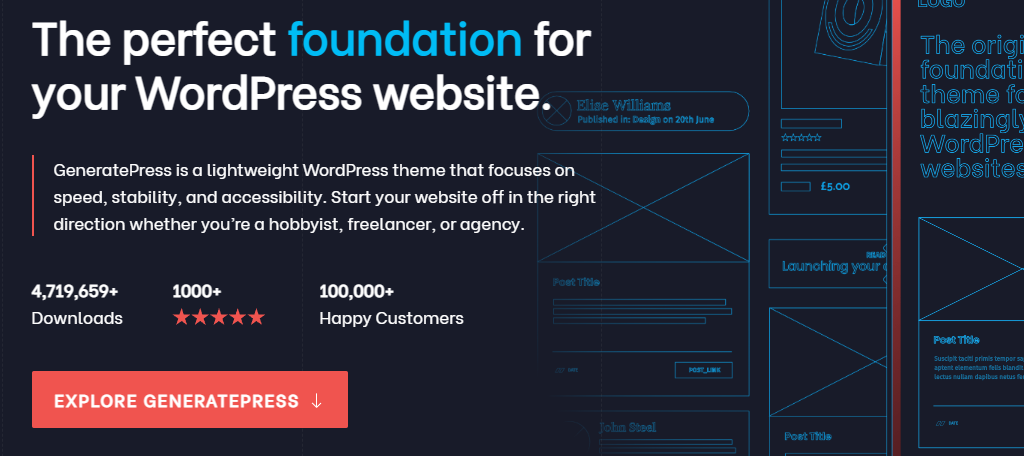**Advertisement for GeneratePress – The Perfect Foundation for Your WordPress Site**

This advertisement appears on the WordPress website, highlighting GeneratePress, a lightweight WordPress theme that emphasizes speed, stability, and accessibility. The central headline reads, "The Perfect Foundation," with "foundation" prominently highlighted. The tagline promotes GeneratePress as the ideal starting point for any WordPress site, suitable for hobbyists, freelancers, and agencies alike.

Key features and accolades of GeneratePress are prominently displayed:
- Over 4,719,659 downloads
- More than 1,000 5-star ratings
- 100,000+ satisfied customers

A call-to-action button labeled "Explore GeneratePress" encourages users to learn more.

Adjacent to the text, the ad features visual elements resembling multiple WordPress website templates. These templates are stylized in a way that makes them look like blueprints, emphasizing the foundational aspect of the theme.

This comprehensive advertisement aims to attract users by showcasing GeneratePress as a reliable and efficient starting point for building a WordPress website.